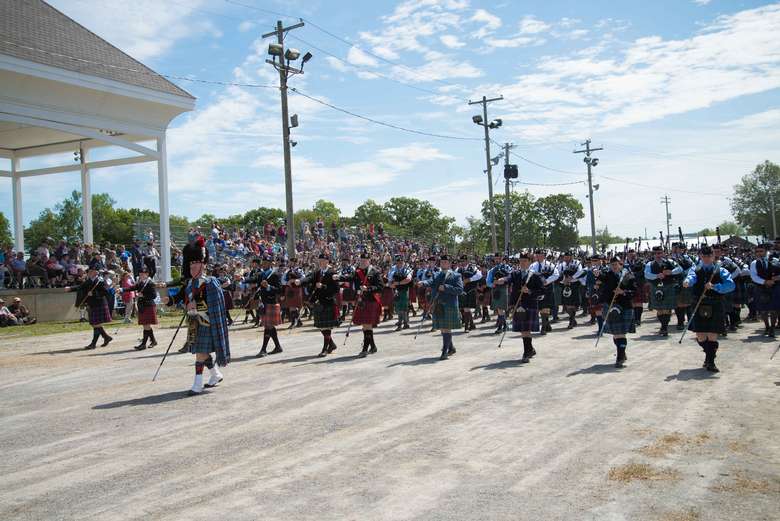The photograph captures an outdoor parade on a beige dirt road under a partly cloudy blue sky. A large contingent of men, all dressed in red and green kilts and tall hats adorned with feathers, march in formation. Many of them are either playing bagpipes or holding staffs. Leading the parade is a single man at the front. Numerous spectators line both sides of the road, some seated on bleachers, while in the left background stands a large gazebo or stage area with an open-sided, roofed top. Telephone poles and a mix of vividly green trees frame the setting, enhancing the lively and festive atmosphere. The parade stretches across the width of the road, contributing to the sense of a grand, musical procession.